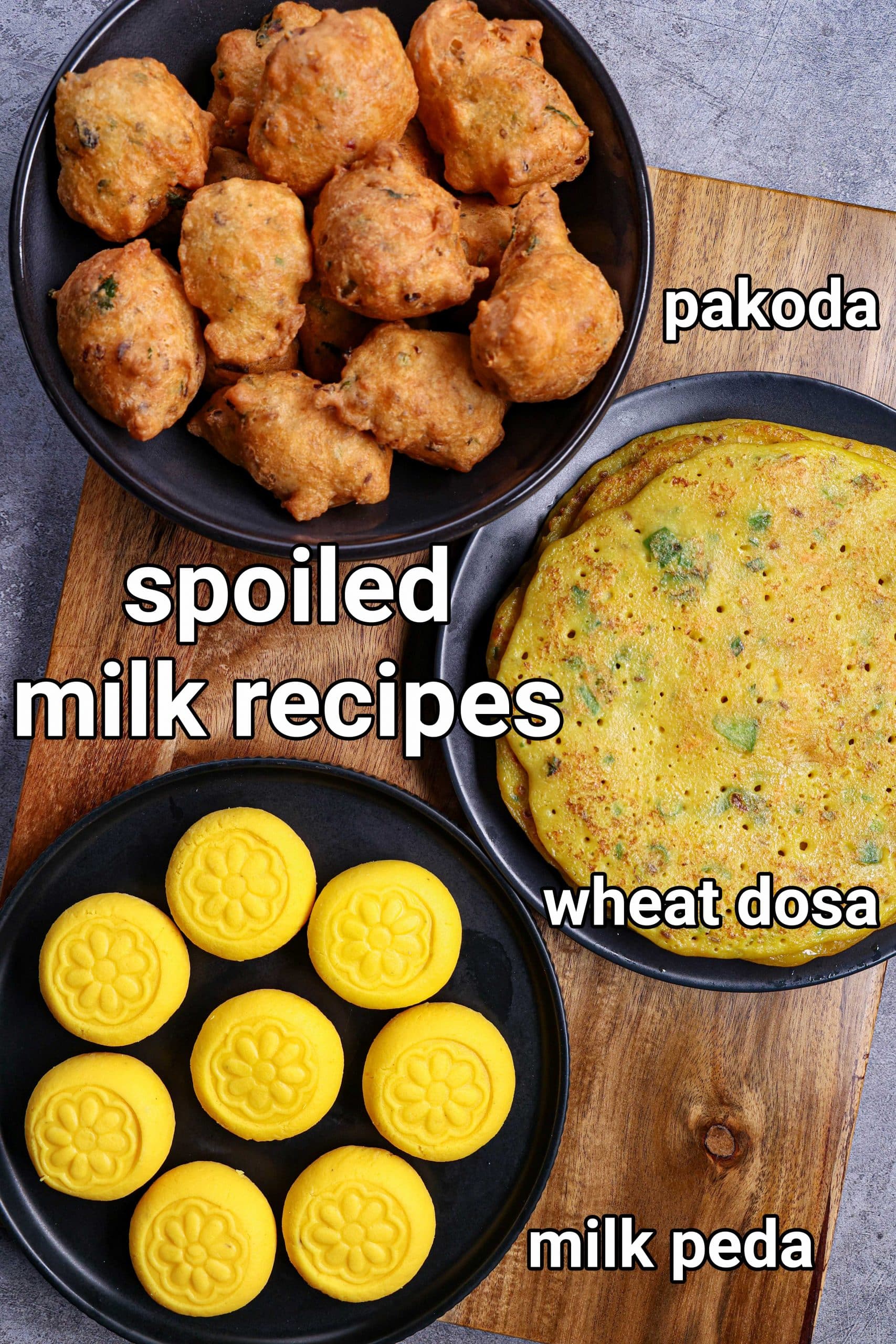The photograph features three black platters arranged on a brown wooden cutting board, showcasing an array of foods labeled as "spoiled milk recipes." In the top-left plate, named "pakoda," there are round, golden-brown, deep-fried items, possibly filled with vegetables or cheese. Adjacent to "pakoda," moving rightward, is a dish labeled "wheat dosa," which looks like a large, savory pancake containing green vegetables, reminiscent of an omelet or quiche. The bottom-left platter, labeled "milk peda," contains circular yellow treats with intricate flower patterns pressed into their centers. The entire arrangement rests on a wooden plank with distinct streaks, possibly placed on a grayish granite countertop, suggesting an indoor setting and hinting at this being part of an advertisement for recipes involving cheese.